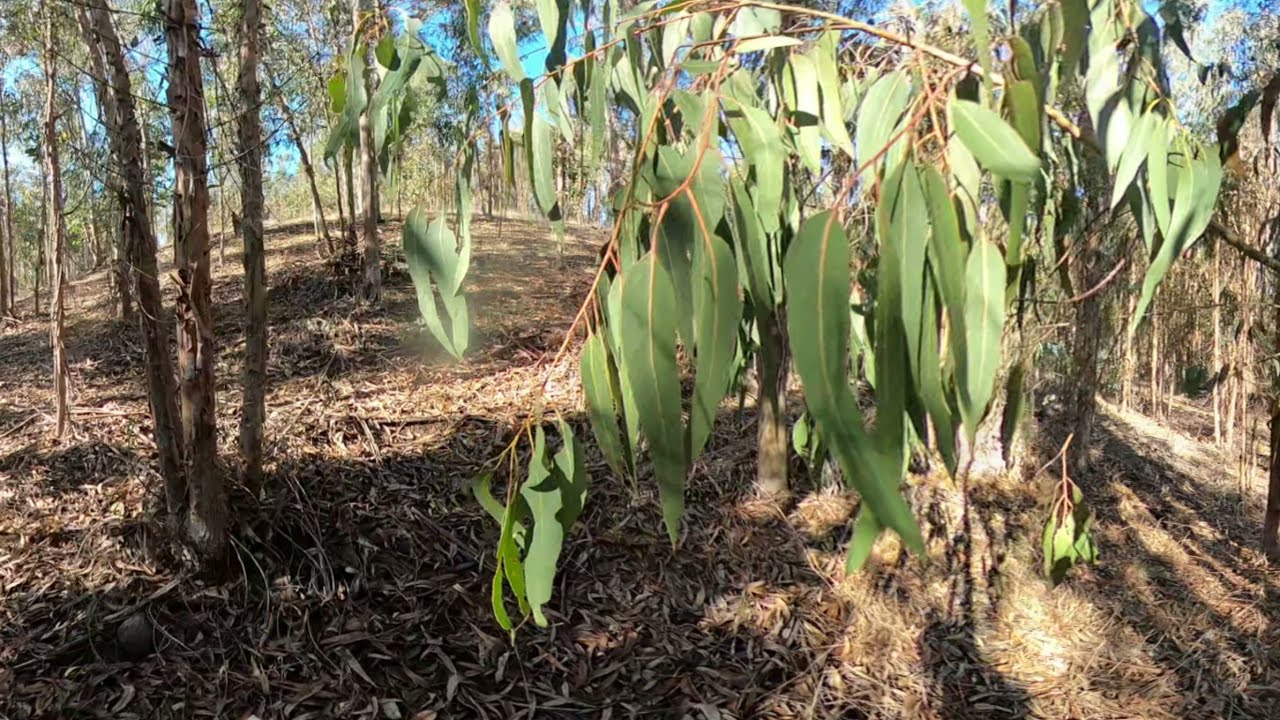The image captures a serene, dry woodland area during the fall, characterized by a ground blanketed with light brown, elongated dead leaves. The sparse trees, mostly leafless, indicate the seasonal transition, while the background reveals patches of bright, cloudless blue sky, illuminating the sun-dappled forest floor. Dominating the center of the photo is a prominent, thin reddish-brown branch hanging at head level, adorned with long, narrow drooping green leaves. This green-laden limb contrasts vividly against the otherwise muted brown surroundings. The scattered sunlight filters through the tree gaps, casting interspersed patches of light and shadow, further enhancing the tranquil, woodsy ambiance of this forest scene.